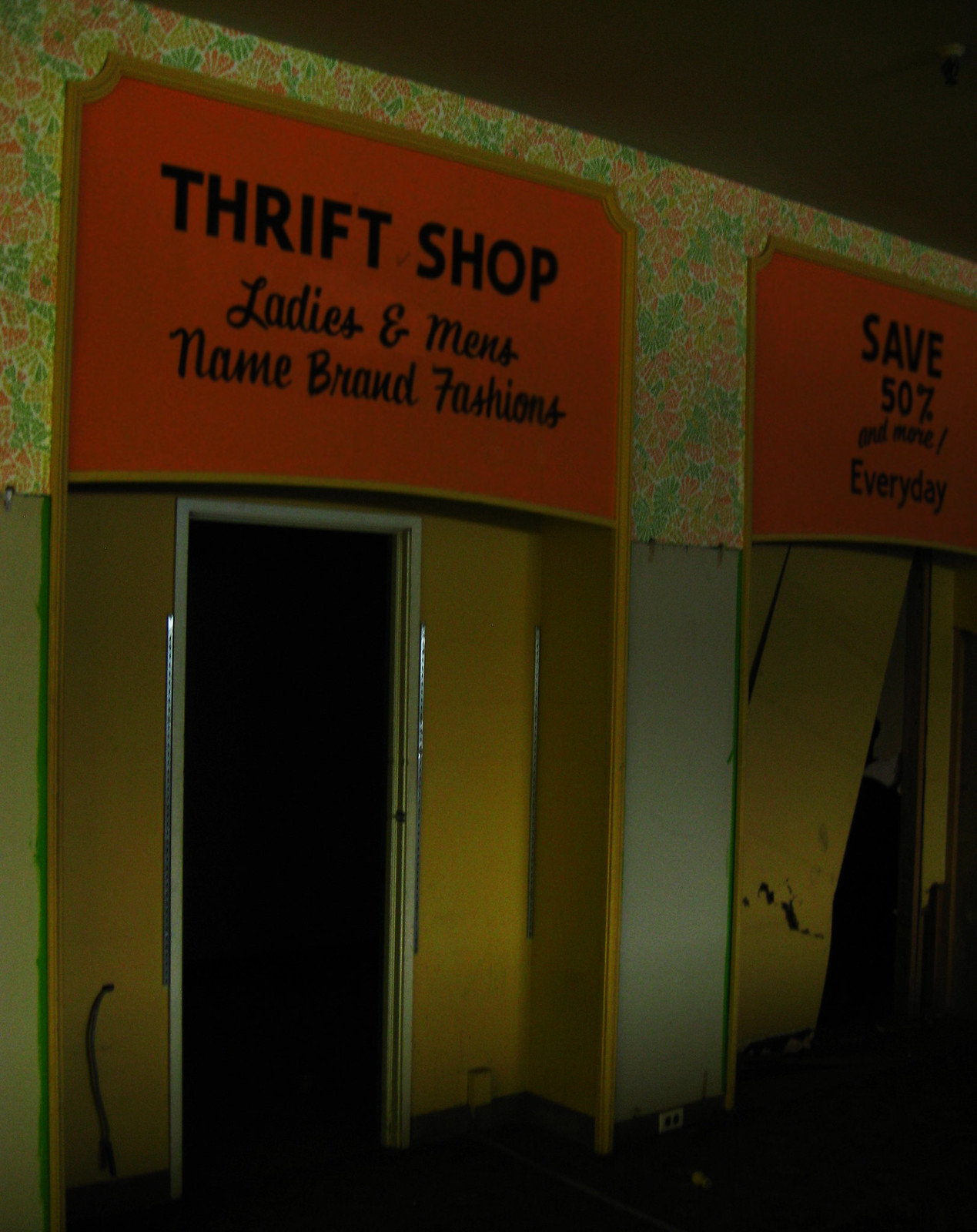This image showcases the entrance of a local thrift shop. Above the single, all-black door, a prominent sign with a red background bears the black lettered inscription: "Thrift Shop - Ladies and Men's Name Brand Fashions." Adjacent to this entrance, the building's façade features walls painted in a dark yellow hue. To the right of the main door, there's another entrance, accompanied by a sign announcing a "Save 50%" promotion, also in black letters. A vibrant, floral-patterned wallpaper in shades of pink and green serves as the backdrop for both signs, adding a splash of color and character to the storefront.